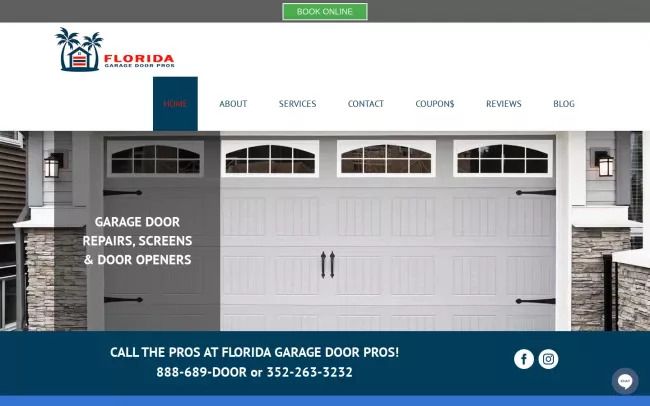The screenshot depicts a website for a garage door service company. At the very top, there is a small, dark gray banner featuring a centered, small green button with white text in all caps reading "BOOK ONLINE." Dominating the center of the website is a photograph of a home's light gray garage door, adorned with black wrought iron features and four arched-top windows with white frames and small panes.

On the left side of the photograph, a translucent gray overlay displays a service offering in white text: "GARAGE DOOR REPAIRS, SCREENS, AND GARAGE DOOR OPENERS." Above the photo, a white banner showcases a clipart image of a house flanked by two palm trees, with red text in all caps reading "FLORIDA." Beneath this, slightly unclear navy blue text seems to state "GARAGE DOOR PACK."

The website includes a navigation menu with several tabs at the top, with the "HOME" tab highlighted in navy blue. The other available tabs are "ABOUT," "SERVICES," "CONTACT," "COUPONS," "REVIEWS," and "BLOG." 

At the bottom of the page, a prominent banner states "CALL THE PROS AT FLORIDA GARAGE DOOR PROS" followed by the phone number, "888-698-DOOR." The banner also features social media links to Facebook and Instagram.